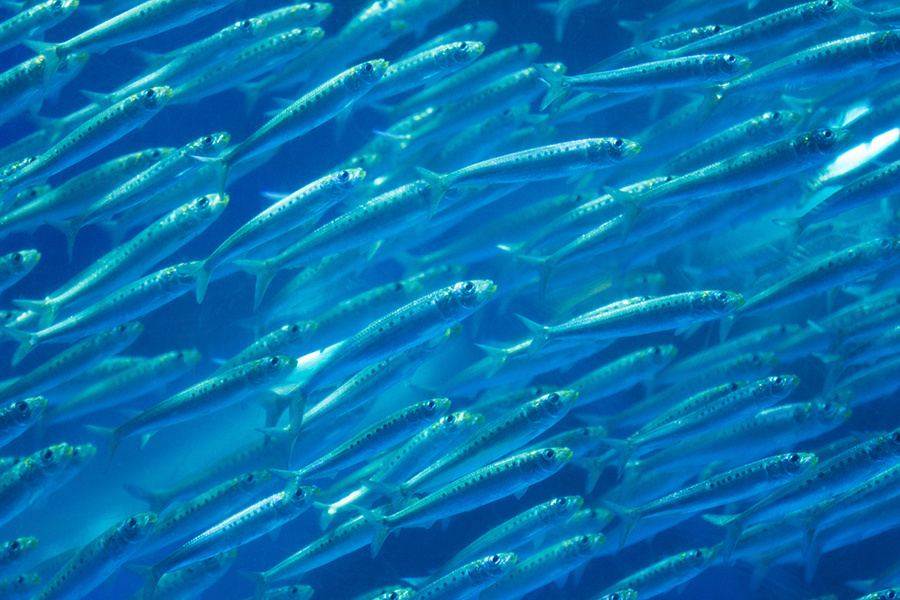Underwater photograph featuring a densely packed school of long, narrow fish swimming diagonally from the bottom left to the upper right corner. The water is a vivid blue, illuminated by hints of sunlight that scatter gracefully throughout the scene. The fish appear to blend with the water, adorned with hues of bluish-green or teal, although they might actually be silvery and just reflecting the ambient blue light. Each fish has distinct dark eyes and small darker dots along their bodies, which shimmer under the light. Despite their small size and delicate appearance with two-pointed tails, the sheer number of fish is overwhelming, forming a tight, cohesive mass. The photograph, wider than it is tall, captures the serene beauty of this underwater spectacle, possibly in an ocean, as the multitude of tiny fish move in unison, creating a mesmerizing display of aquatic life.